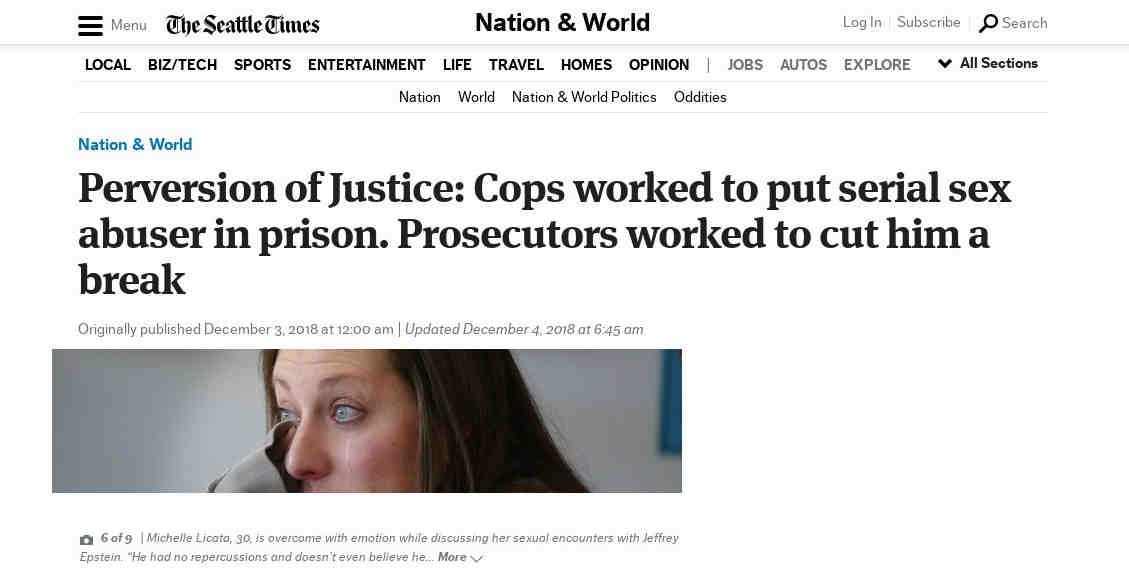Screenshot of a Seattle Times webpage featuring a detailed article. The webpage has a dark header with "menu" and a three-bar icon on the top left, followed by "The Seattle Times" logo. The header includes several navigation options: "Nation & World" in the middle, "Subscribe," "Search" with a magnifying glass icon. Beneath the primary header, there is a secondary navigation bar listing categories like Local, Biz/Tech, Sports, Entertainment, Life, Travel, Homes, Opinion, Jobs, Autos, and Explore, with an arrow indicating all sections.

The article is categorized under "Nation & World" and titled: "Perversion of Justice: Cops Work to Put Serial Sex Abuser in Prison, Prosecutors Work to Cut Him a Break." It was originally published on December 3, 2018, at 12:00 AM and updated on December 4, 2018, at 6:45 AM.

The article features an image partially cut off, depicting a woman crying. The caption reads: "6 of 9 Michelle Lakata, 30, is overcome with emotion while discussing her sexual encounters with Jeffrey Epstein. He had no repercussions and doesn't even believe he..." The woman has blue eyes, brown hair, and is wiping away tears with the sleeve of her sweater or shirt. The background is white with black text.